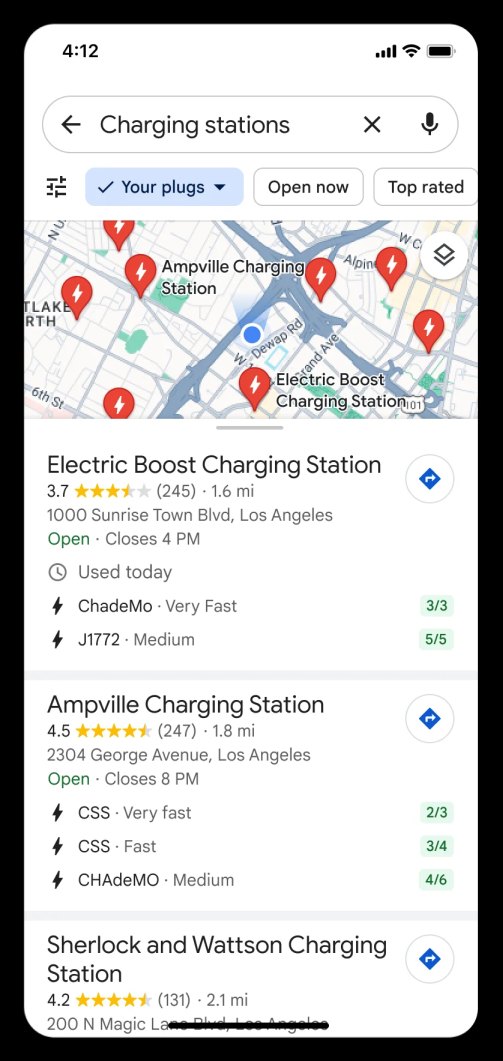This is a screenshot depicting a Google search results page for charging stations. The interface features a search bar at the top, with various filter buttons beneath it. The available filters include "Plugs," "Open Now," and "Top Rated," with the "Plugs" filter currently highlighted in light blue and marked with a checkmark. Below the filters, a partial map is visible, displaying several red map pins indicating the locations of different charging stations.

Three specific search results are presented sequentially. The first result is titled "Electric Boost Charging Station." Each result includes a title, the name of the station, and a brief overview represented by store reviews. To the right of the store names, there is an arrow icon that can be clicked for directions. Further details about each station are provided beneath the titles, including the address, opening times, charge speed, and user ratings. The ratings are visually denoted by green text to the right of the information.